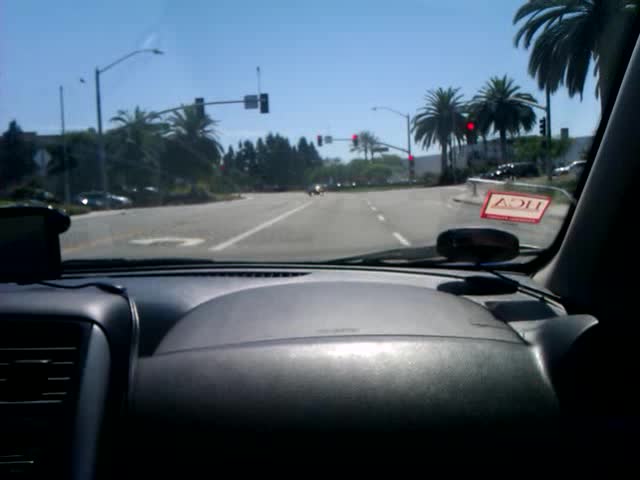The photograph, taken from the perspective of a car's passenger seat, showcases the inside of the car, particularly the black dashboard. A sticker is visible on the windshield's right side; it is red and white in a rectangular shape and possibly reads "UCA" or "HGA." Mounted on the dashboard is an unidentified device with a cable emerging from it, possibly a dash cam or radar detector. Through the windshield, the scene features a wide, multi-lane road stretching out towards an intersection. The road has two lanes in each direction, a central turning lane, and all the traffic lights at the intersection are red. The intersection is flanked by streetlights and substantial overhead traffic lights suspended from poles. On both sides of the street, a row of palm trees lines the landscape, resilient and large in stature. In the distance, the top of a mountain can be glimpsed on the upper right portion of the image beneath a clear, bright blue sky, adding depth to the day's serene atmosphere. Some cars are visible in the far lanes, hinting at approaching traffic.